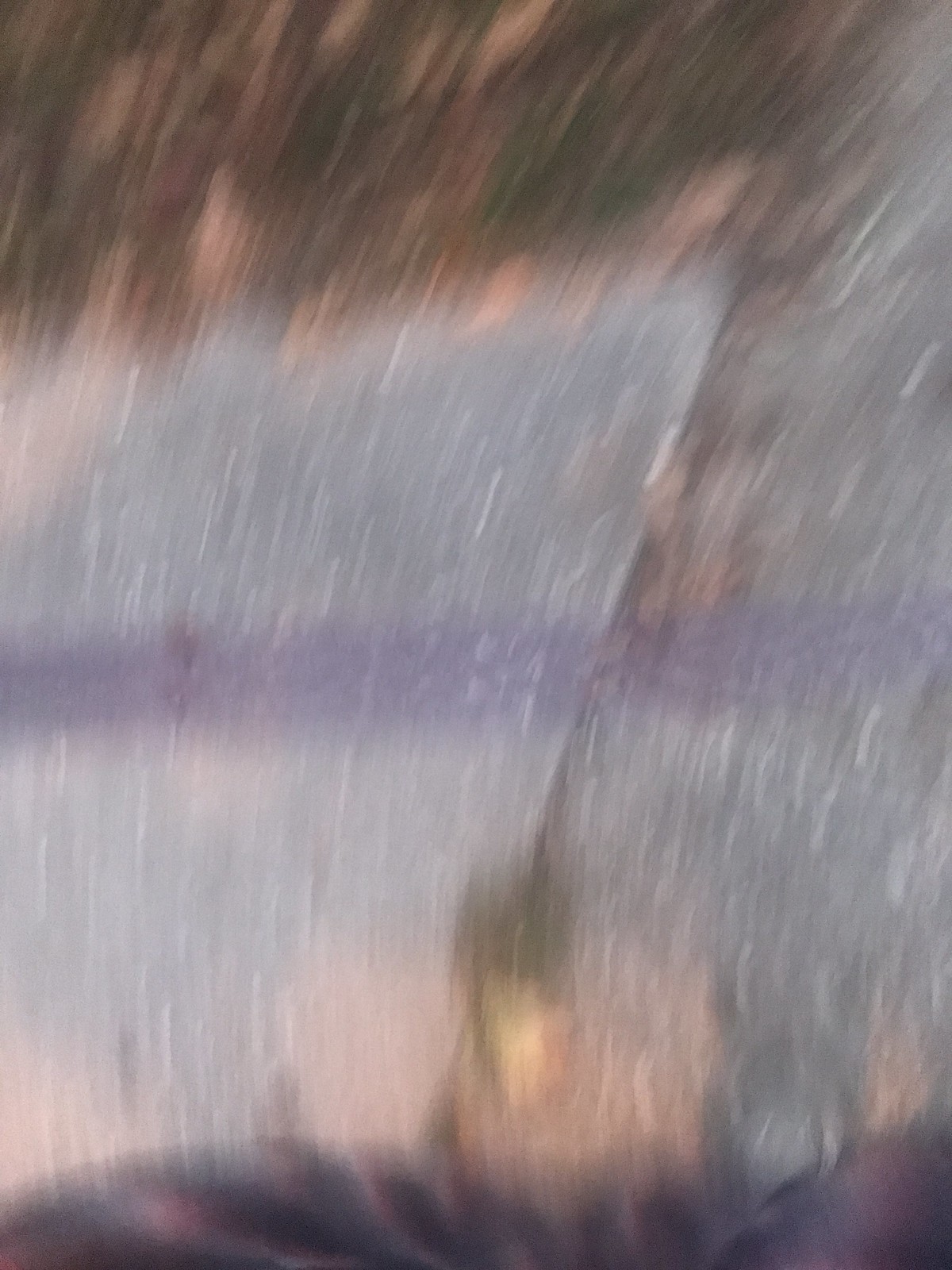The extremely blurry image is dominated by motion and distortion, making it difficult to discern any specific objects or figures. However, certain elements are vaguely noticeable: a shiny, rain-soaked surface, possibly a tall road or sidewalk, appears to reflect various light sources. You can spot scattered white dots, patches of red light, and streaks of a purplish hue across the image. A large yellow light is visible at the bottom, contributing to the reflective quality. The overall picture hints at the reflection of lights on a wet surface, amidst potential camera movement. Sparse details suggest a darker hue at the bottom, transitioning to lighter blue in the center, and dark again towards the top. Orange and brown tones indicate possible autumn leaves scattered on what could be a stone or cement sidewalk, albeit blurry. No clear objects, text, or well-defined figures are discernible, with the image overall remaining highly ambiguous and out of focus.